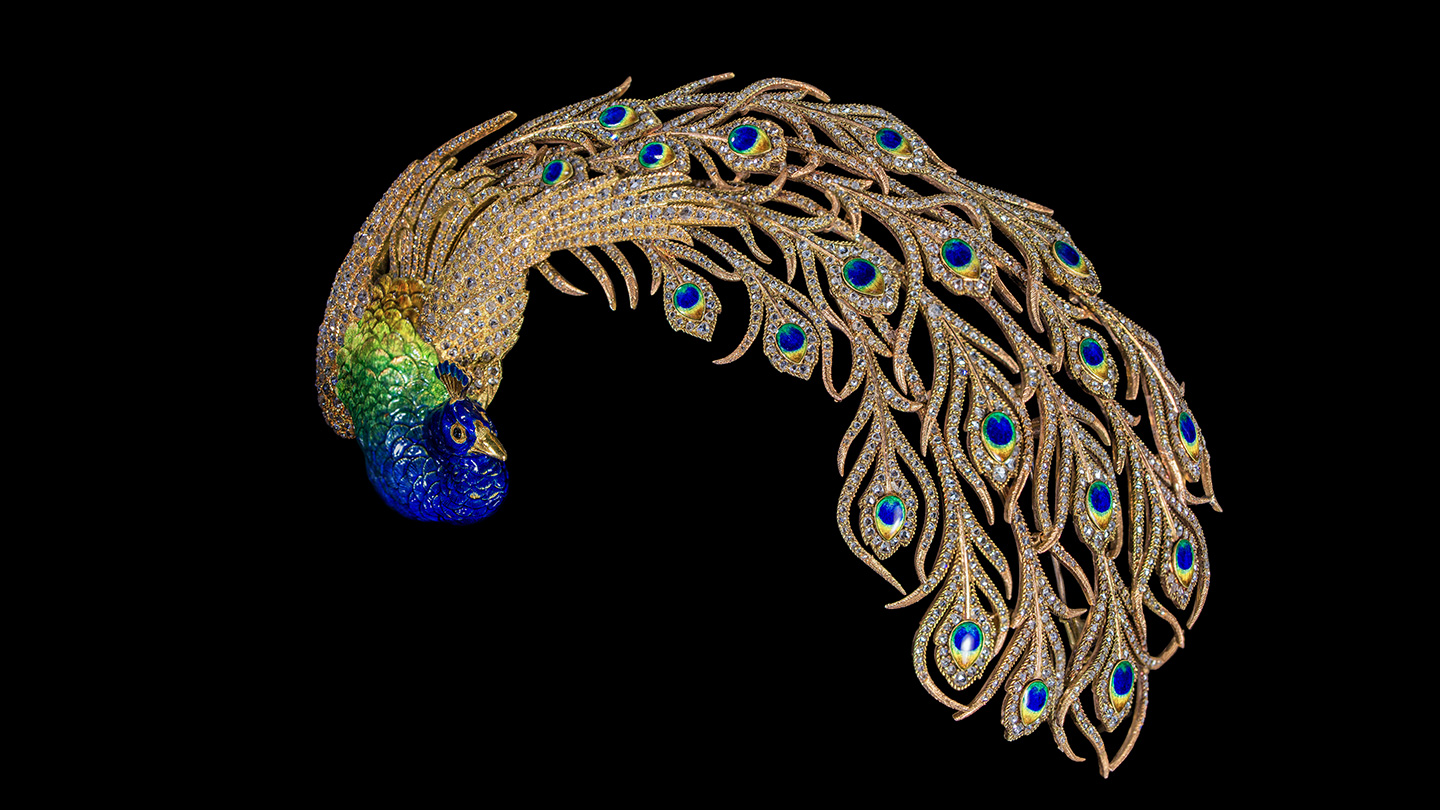This detailed and ornate brooch features a peacock with a royal blue body and head, complemented by a golden beak and eyes. Its vibrant plumage transitions from green and yellow gradients into an elaborate tail. The tail spirals clockwise to the right and is substantially larger than the body, appearing to be about five times its size. Encrusted with hundreds of small diamonds and intersected by dark blue spots resembling sapphires, the tail culminates in a diamond-shaped end adorned with intricate swirls and sparkling white stones. The luxurious design of the brooch makes it a striking piece of jewelry, with its rich blend of colors and gemstones creating a captivating visual effect.